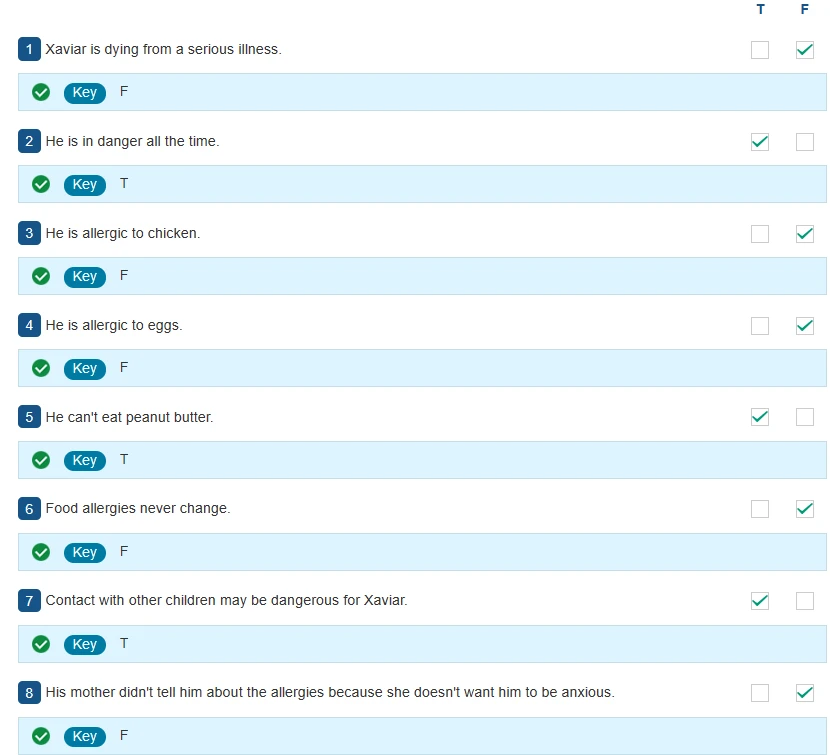The background of the image features an alternating pattern of white and light blue stripes. This striped pattern runs horizontally across the page. In the top portion of the image, there's a white section on the right-hand side containing a bold letter "T." The content is organized into two columns labeled "True" and "False" in blue text.

The image displays several rows, where each row provides a statement and two corresponding boxes under "True" and "False." The statements pertain to a character named Xavier and his health conditions and experiences. Next to each statement, a green checkmark indicates the user's response, and below the statement, the correct answer (key) is provided in blue text.

1. "If Xavier is dying from a serious illness":
   - User response: False (Green check here)
   - Key answer: False

2. "He is in danger all the time":
   - User response: True
   - Key answer: True

3. "He is allergic to chicken":
   - User response: False (Green check here)
   - Key answer: False

4. "He is allergic to eggs":
   - User response: False (Green check here)
   - Key answer: False

5. "He can't eat peanut butter":
   - User response: True (Green check here)
   - Key answer: True

6. "Food allergies never change":
   - User response: False (Green check here)
   - Key answer: False

7. "Contact with other children may be dangerous for Xavier":
   - User response: True (Green check here)
   - Key answer: True

8. "His mother didn’t tell him about the allergies because she doesn’t want him to be anxious":
   - User response: False (Green check here)
   - Key answer: False